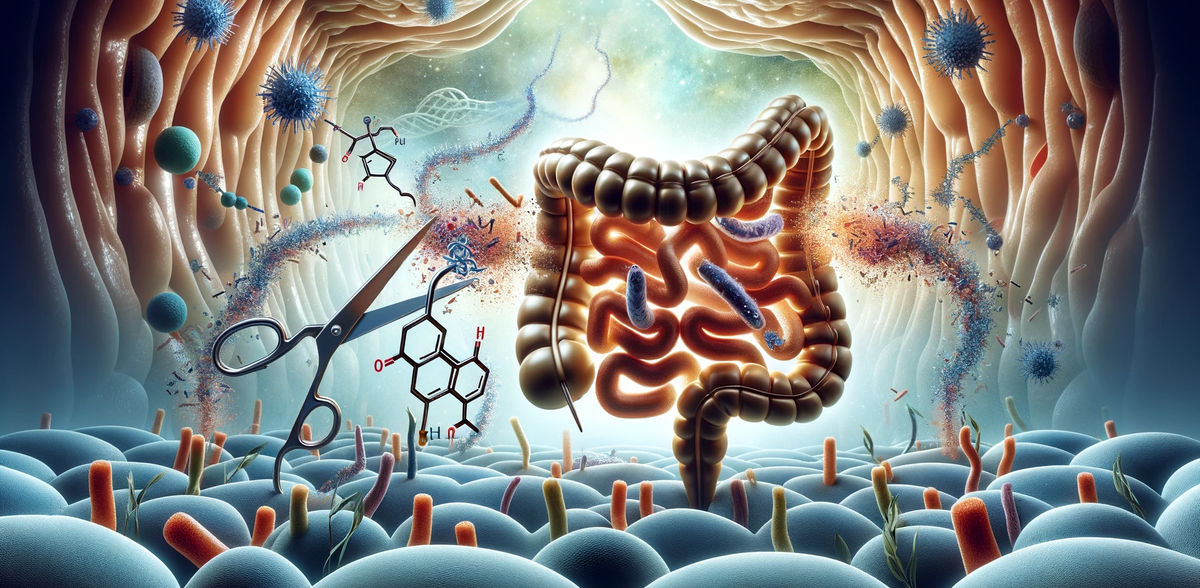The illustration portrays a graphic, well-detailed, and somewhat unsettling depiction of the interior of a human body, focusing prominently on the intestines. Rendered in bright, primary colors such as purple, blue, and pink, the image showcases the intestines winding up, over, and down, interspersed with other smaller intestinal segments. To the left and slightly above this central structure, there's a depiction of DNA or molecules being cut by a pair of scissors, with severed strands floating upwards.

The top section of the image resembles a tunnel encasing this visceral scene, suggesting an immersive view inside the body. Various round, smushy, and squishy elements are present, enhancing the biological atmosphere. The image is populated with diverse details: spiky blue bacteria, protodines, visible atoms, molecules, and even what appear to be germs and other microscopic particles in shades of orange, purple, green, and yellow. Aqua green circular entities float around, alongside vein-like structures and protein-like constructs, contributing to a chaotic yet detailed visualization of the body's interior workings. Overall, it’s a disturbing yet intricately designed portrayal of human anatomy, blending artistic creativity with biological elements.